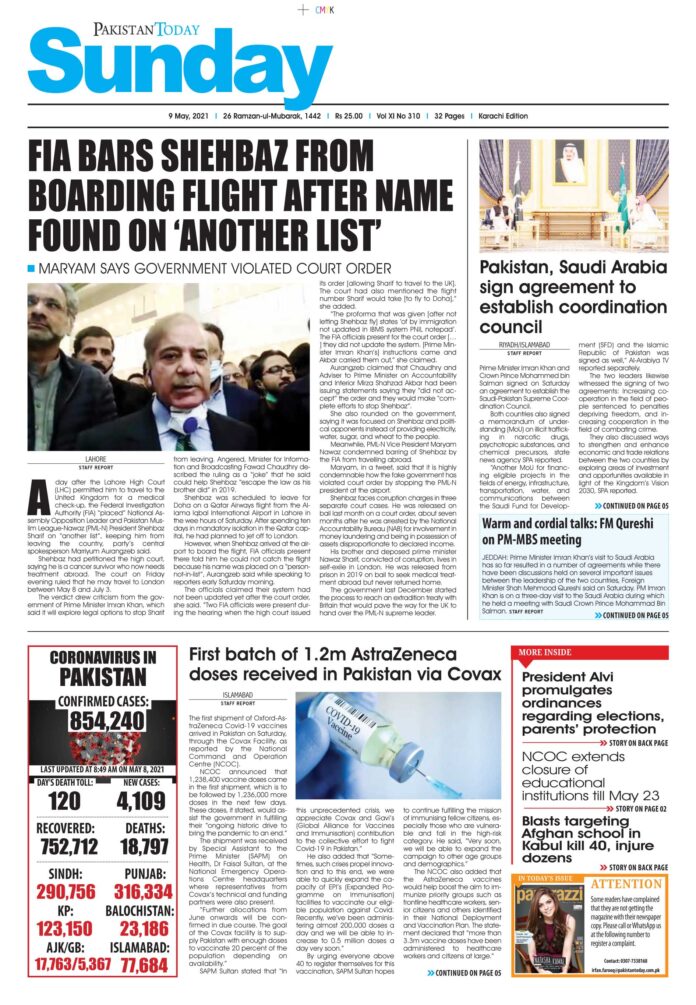The image portrays a detailed newspaper page from "Pakistan Today," designed in a traditional print format with distinct sections for each article. At the top, the headline in large blue text reads "Sunday," and just below that, the masthead prominently displays "Pakistan Today" along with a partially legible date, likely from 2021. The layout mirrors that of a conventional broadsheet newspaper, with articles organized in square and rectangular blocks of varying sizes.

The upper section of the page features the lead article titled "FIA bars Shabazz from boarding flight after name found on 'another list'," accompanied by a subheading stating "Merriam says government violated court order." The article includes a photograph of an older man in a suit, standing among a group of taller men. Adjacent to this, another headline reads "Pakistan, Saudi Arabia sign agreement to establish coordination council," indicating key diplomatic developments.

The bottom half of the page is divided into three additional sections, one of which prominently features an infographic detailing the impact of the coronavirus pandemic in Pakistan. The overall design emphasizes a traditional newspaper's aesthetic, blending textual content with visual elements for comprehensive reportage.